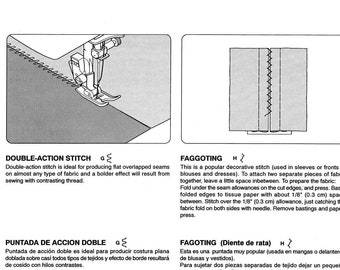This image, likely an excerpt from a sewing machine manual, features a meticulously structured, formal instructional design. Digitally created in black and white, the illustration consists of two main graphics accompanied by text blocks in both English and a European language, possibly German or Spanish, providing direct translations.

The left section showcases a rectangular illustration titled "Double Action Stitch," depicting the head of a sewing machine performing the stitch, which is described as ideal for producing flat overlap seams in nearly any fabric, with a bolder effect achievable using contrasting thread. Below the title, the text details these instructions in both English and its translated counterpart.

On the right, the illustration labeled "Faggoting" features a zigzag stitch, with the term "faggoting diente de rata" provided in translation. Similarly structured, the title is followed by explanatory text in smaller font, outlining the stitch's characteristics in both languages. Each section includes bolded headings above the detailed descriptions, offering readers a comprehensive guide to these specific sewing techniques.